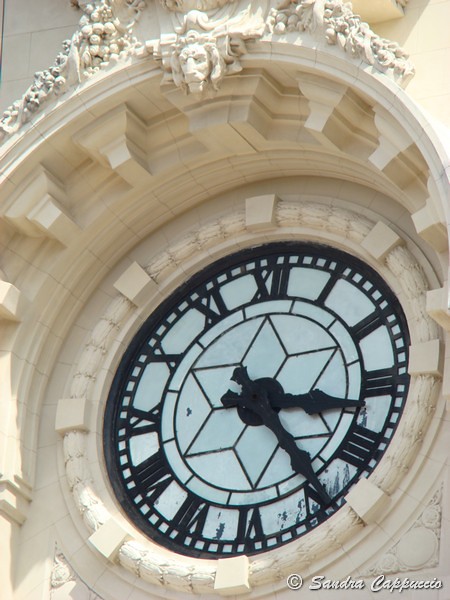The image depicts an outdoor color photograph taken during the day, looking up at the ornate facade of a Renaissance-style building made of lightly colored stone. Central to the image is a fancy, glassy clock recessed into the lower half of the wall, featuring a white face with black Roman numerals and hands. The small hand points near 3, while the large hand points just before 5, indicating a time of 3:25. Surrounding the clock is intricate stonework, including white concrete arching and ornate designs. Above the clock, an extravagant archway culminates in a capstone bearing a lion’s head, slightly angled to the left, and surrounded by fruit-like circular objects. The bottom right of the clock face shows an overlay text reading "© Sandra Cappuccio." The bright, natural daylight enhances the sharpness and focus of the photograph.